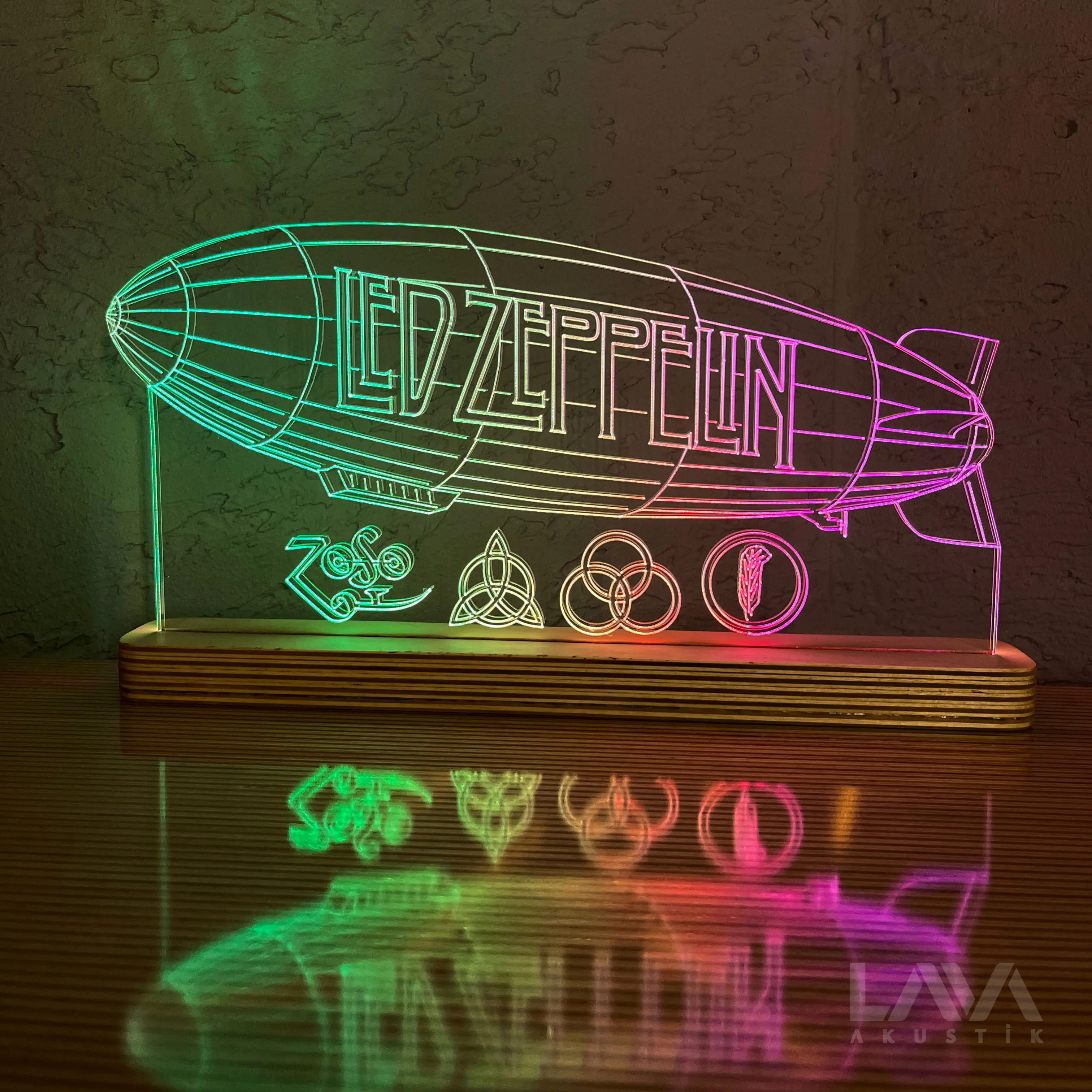The photograph captures a detailed indoor scene centered on a glass-topped table. Set against a rough-textured wall, the table holds a striking decorative item: a neon light sculpture of the Led Zeppelin blimp. This sculpture features a nearly rectangular golden bronze or wooden base and presents a glass design emitting light. The blimp, which is oriented towards the left, illuminates with a green front and purple rear. The name "Led Zeppelin" is prominently displayed in green and purple lights on the blimp, while four famous Led Zeppelin symbols, including "Zozo" from the Led Zeppelin III album, are displayed nearby. The reflective surface of the table mirrors the vivid colors and intricate details of the blimp, enhancing its visual impact.